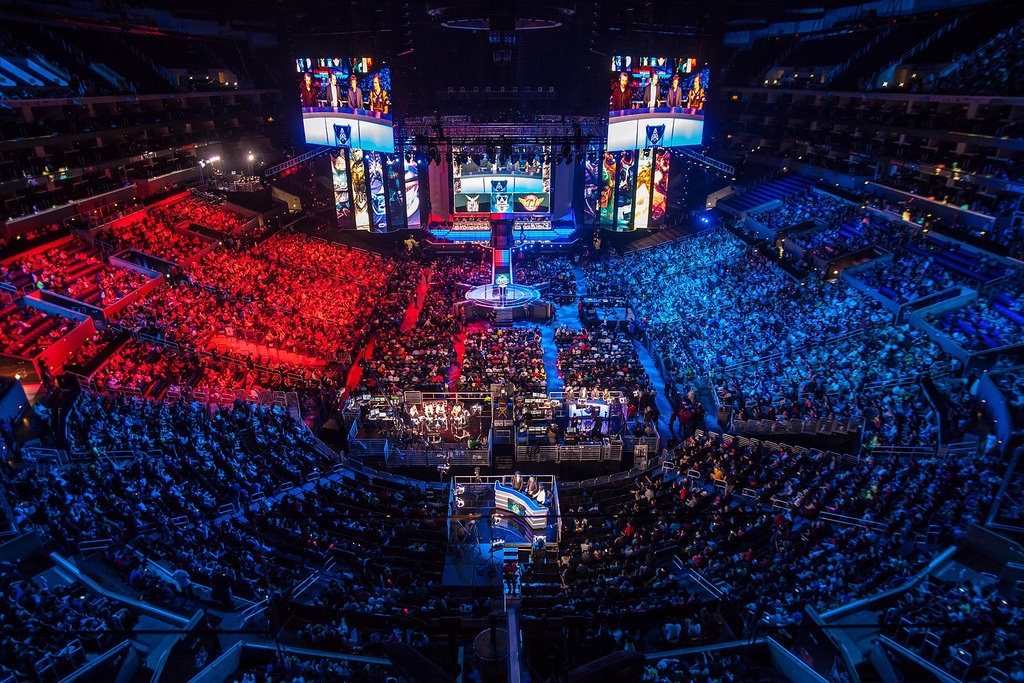The photograph is a high-resolution, full-color image capturing the vibrant and electrifying atmosphere of an indoor eSports event taking place in a massive stadium. The arena is packed with hundreds, if not thousands, of spectators, whose seating areas are highlighted with distinct colors: red on the left, blue on the right, and darker blue at the front of the image, creating a visually striking contrast. 

At the center of the rectangular-shaped arena is a prominent stage, showcasing several huge monitors and display screens. Two large TVs hang on either side of the stage, each displaying the same image of four people seated at a desk, presumably the broadcasters. Another large screen is positioned at the back of the stage, completing the immersive setup for the event. Additional monitors adorn the back wall, enhancing the spectators' viewing experience.

The lighting within the stadium is predominantly blue, lending a cool, dynamic feel to the scene, except for the upper left portion, which is distinctively bathed in red light. This difference in lighting further accentuates the specific areas designated for spectators.

On the screens flanking the main stage, images of video game characters are prominently displayed, indicating the eSports nature of the event. In front of these screens, the players, intensively focused, can be seen at their computers, immersed in their games. The crowd, filling nearly every available seat, adds to the palpable excitement in the air, making it a thrilling depiction of a large-scale eSports gathering.